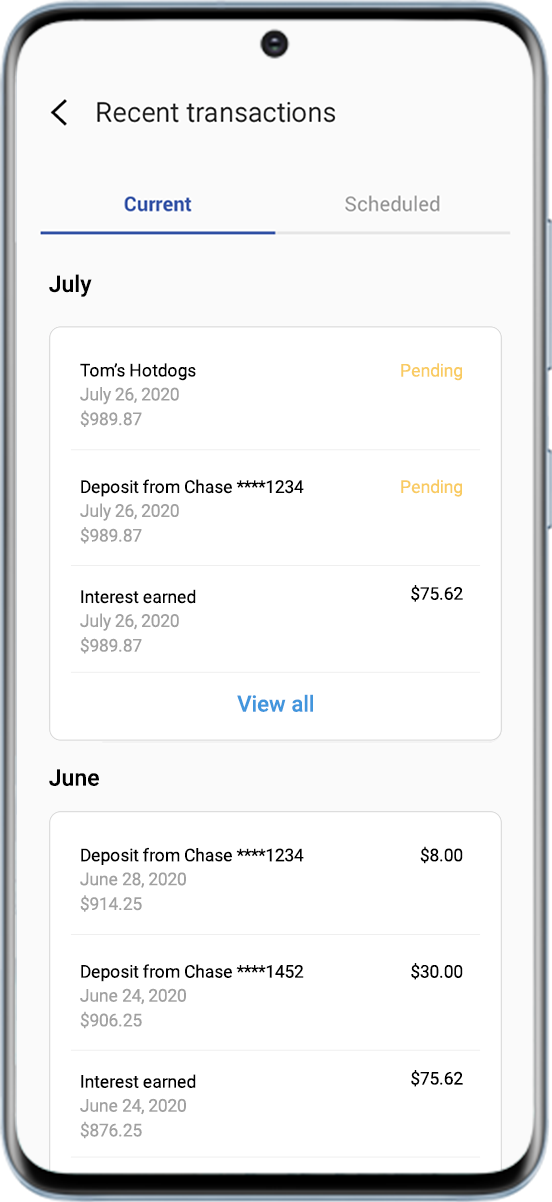The image features a likely iPhone displaying a banking app on its screen. The phone has a black rim, while the app interface is predominantly white. At the top center of the screen, there is a scroll button. Below it, the text "Recent Transactions" is displayed in black font with a back arrow beside it. Underneath this heading, there are two tabs: "Current" and "Scheduled." The "Current" tab is active, highlighted in blue and underlined in blue, whereas the "Scheduled" tab is inactive and grayed out.

The screen then shows the heading "July," followed by a bright white box listing three transactions. In the center of this box, there is a blue-font option labeled "View All." The transactions listed under July are:

1. **Tom's Hot Dog** on July 26, 2020, for **$989.87**, marked as pending in a yellow tangerine font.
2. **Deposit from Chase**, account ending in **1234**, also pending on July 26.
3. **Interest Earned** on July 26, amounting to **$75.62**.

Following the July transactions, there is the heading "June" with another bright white box listing three transactions:

1. **Deposit from Chase**, account ending in **1234**, for **$8** on June 28, 2020.
2. **Deposit from Chase**, account ending in **1452**, for **$30**.
3. **Interest Earned** on June 24, amounting to **$75.62**.

The detailed listing provides a clear view of the recent financial activities and balances within the app, with notable emphasis on the pending transactions and interest earned for both months.